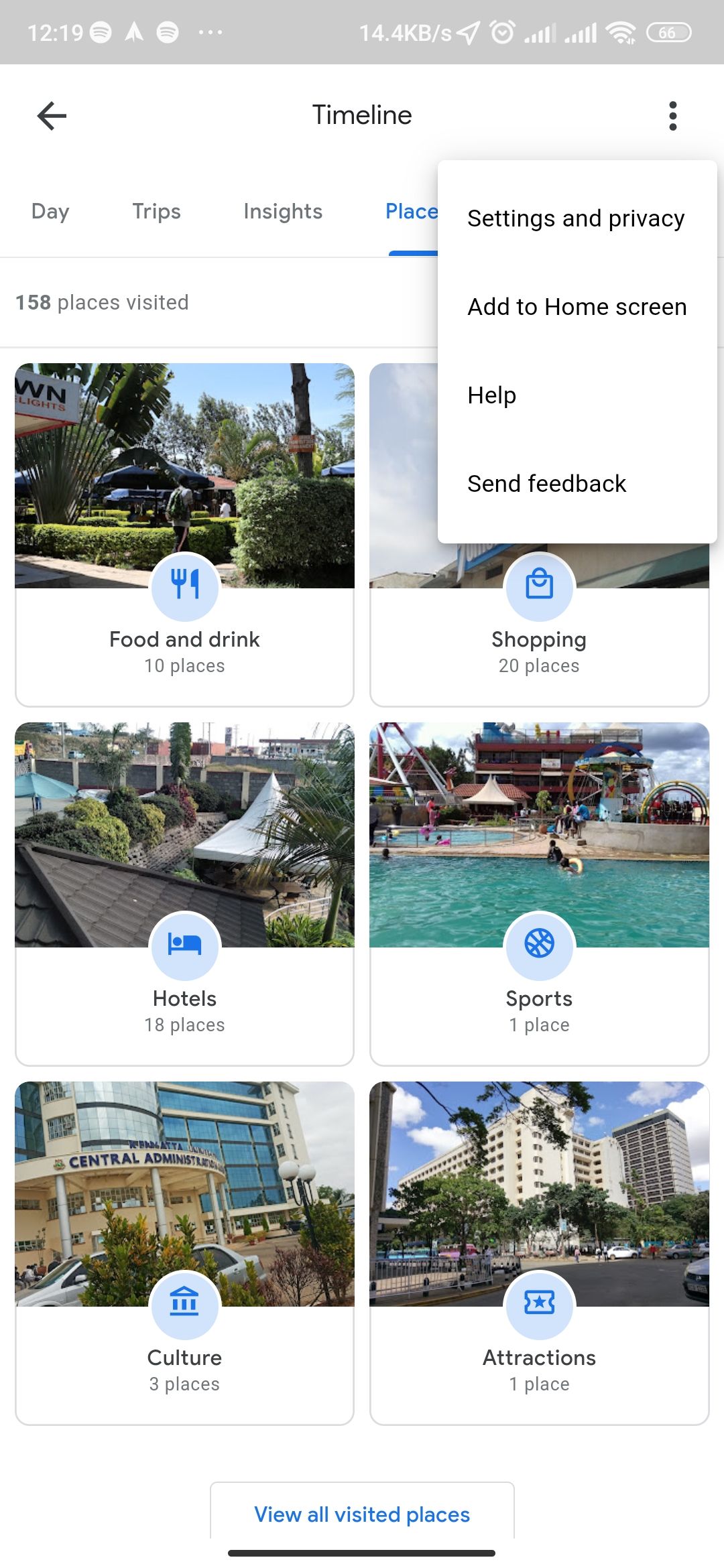The image is a screenshot from a digital platform displaying various user metrics and navigation options. At the top, the screen shows a status bar with indicators for battery life, connectivity, and the current time, which is 12:19. Directly beneath this, the word "Timeline" is prominently displayed in black text with a leftward arrow, followed by menu options labeled "Day Trips," "Insights," and "Places." The "Places" option is highlighted in blue, indicating it is currently selected.

A pop-up menu is overlaid on the screen, containing options for "Settings and Privacy," "Add to Home Screen," "Help," and "Send Feedback." Below this pop-up, the main content shows a summary of 158 places visited, accompanied by thumbnail images representing different categories of places.

The categories include:
1. Food and Drink – 10 places, depicted with a relevant photograph.
2. Shopping – 20 places, partially obscured by the pop-up menu.
3. Hotels – 18 or 19 places, shown with an illustrative image.
4. Sports – 1 place, also accompanied by a related photograph.
5. Culture – 3 places, with its respective image.
6. Attractions – 1 place, visually represented.

At the bottom of the main section, there is a blue button labeled "View All Visited Places," arranged within a bounding box. Beneath this section, a black line demarcates the end of the visible information, signifying that no additional content follows.